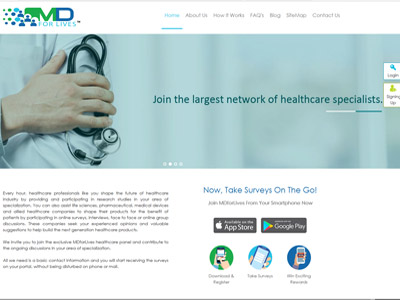This is a detailed description of a website's homepage screenshot:

The homepage features a white background above a white header located at the top of the page. On the left side of the header, there is a logo comprising the letters "MD." The "M" is green with a green box attached to its left side, while the "D" is blue. Below the logo, the phrase "4 Lives" is written in light blue text, accompanied by icons of people in blue on its left. To the left of the icons, multicolored dots in varying shades of blue, dark blue, and green gradually diminish in size as they extend leftward.

To the right of the logo and tagline, a navigation menu is displayed. The first option, "Home," is highlighted in light blue text with a matching underline to indicate its selection. The subsequent sections, in gray text, include "About Us," "How It Works," "FAQs," "Blog," "Sitemap," and "Contact Us."

Directly below the header, a full-width photograph serves as a background image with overlaid text. The photograph has a greenish-blue tint and depicts a close-up view of a hand, originating from the left side of the frame, placed on the wrinkled fabric of a doctor's coat while holding a stethoscope to an arm. Blurred white curtains are visible in the background. Superimposed on this image, the text "Join the Largest Network of Healthcare Specialists" appears in blue.

At the bottom of this image, there are four navigational dots indicating the current position within the slideshow. The first dot is light gray, the second dot is white (indicating the active slide), and the third and fourth dots are light gray. Additionally, two white tabs featuring colorful icons are positioned towards the upper right corner of the image.

Below the photograph, towards the lower-left side of the page, are three paragraphs of text, which are unfortunately too blurry to be legible.